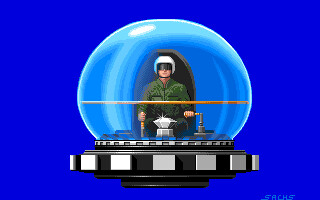In this retro-styled computer game, the image showcases a character dressed in a green military-like pilot's outfit and a white helmet adorned with dark sunglasses. The character is seated in a dome-shaped vehicle featuring a crystalline bubble canopy. He grips two controls, steering the vehicle with purpose. Directly in front of him, a sparkling silver diamond rests elegantly on a square pedestal. The base of his spaceship is rounded, featuring a sleek silver trim with a black underside. The background sky is a brilliant, cloudless blue, enhancing the vividness of the scene.